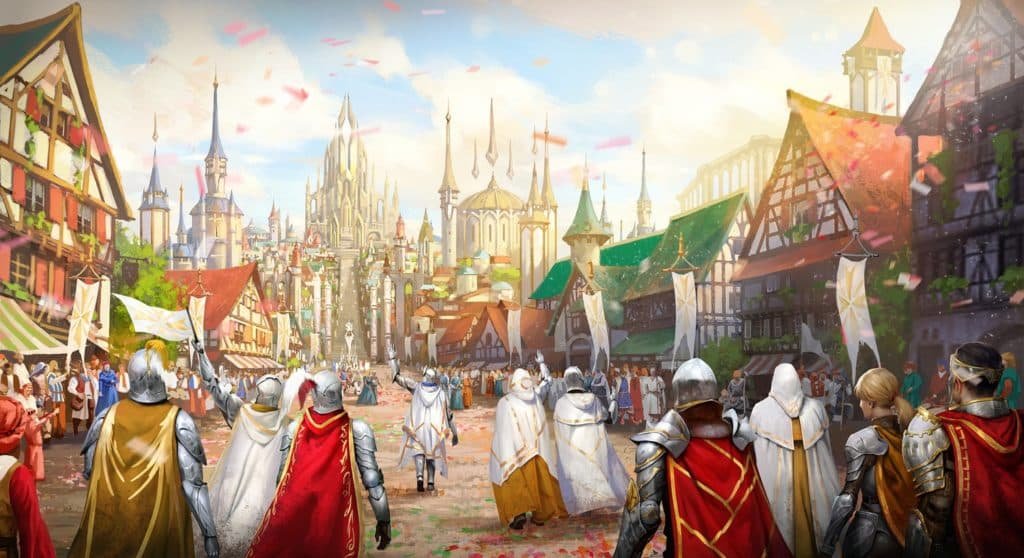The painting depicts a medieval scene with a group of knights, seen from the back, walking down a central pathway flanked by Tudor-style houses and various businesses. These buildings, likely bars and shops, line both sides of the street, where townspeople can be seen greeting the knights. The knights are adorned in silver armor, with some wearing assorted capes – predominantly red, with a notable gold cape and a white cape worn by the leading knight who has his left hand raised, possibly signaling or leading the rest. The scene suggests these knights could be returning from battle or participating in a parade, moving towards a distant large castle whose spires are visible under a light blue sky with wispy clouds and flags flying.